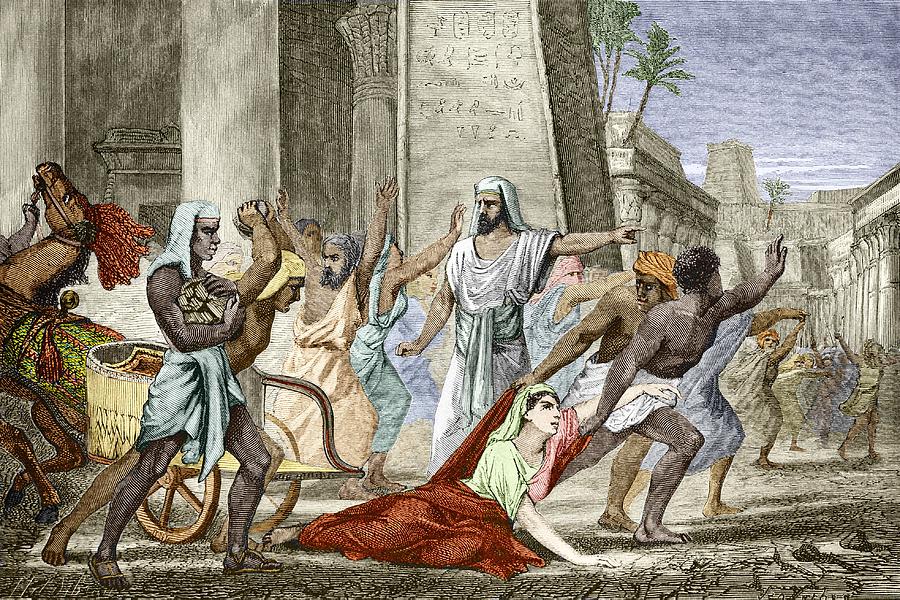The painting vividly portrays an ancient Roman or Greek-inspired scene. Dominating the top right of the image, beige buildings reflect the era's architectural style, punctuated by a grayish-blue sky and two bright green palm trees growing from a rooftop. Horizontally across the middle, numerous figures appear in motion, heading from left to right, their gazes fixated leftwards as if fleeing from something unseen. They are clad in toga-like garments, emulating ancient civilian wear. Among them, a lady in a red dress with a green top lies prostrate on the ground, being dragged by two dark-skinned men, suggesting a conflict. Adjacent is a commanding white man, arm outstretched, directing with authority. An animated horse rears nearby, its brown body accented by a bright green saddle and a beige basket. The lower third of the painting reveals a textured, crumbled mud-like stone surface, harmonizing with the buildings' beige hue. The composition exudes an atmosphere of ancient turmoil and urgency.